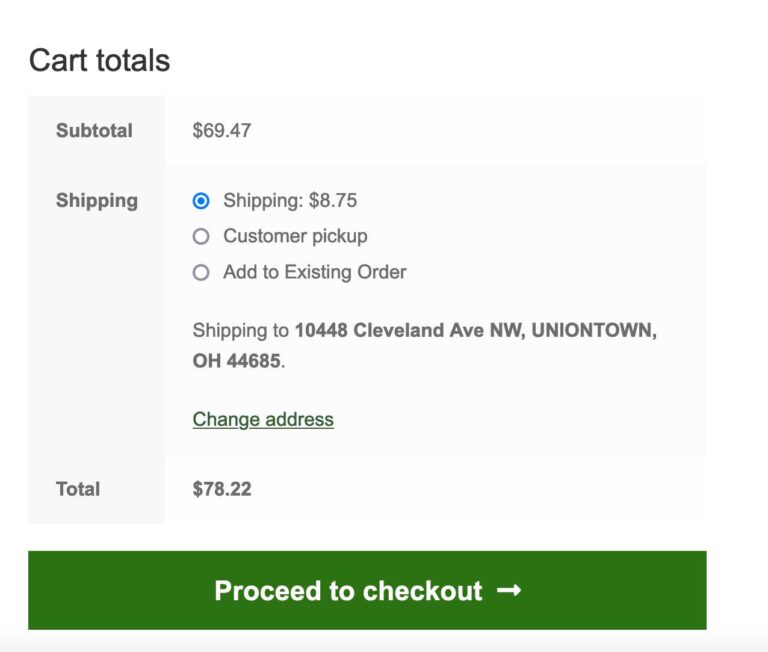Screenshot titled "Cart Totals"

Subtotal: $69.47  
Shipping Fee: $8.75  
Shipping Method: Checked for shipping to 10448 Cleveland Avenue, Northwest, Uniontown, Ohio, 44685  
Additional Options: Customer Pickup and Add to Existing Order (unchecked)  
Address Modification: Option available to change the address  
Order Total: $78.22  

A visually appealing sage green bar at the bottom of the screen prompts users to "Proceed to Checkout," accompanied by a directional arrow indicating the next step in the process. The cart interface is clear and user-friendly, displaying all essential information apart from the actual items purchased.